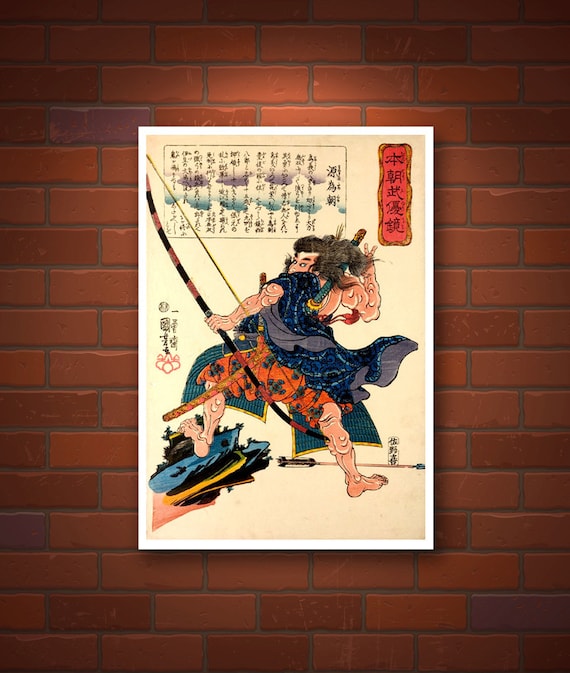The image depicts a detailed drawing of a poster on a brick wall. The bricks vary in shades of red and purplish hues, providing a textured backdrop. The poster itself has a clean white border encompassing a light yellow background. Prominently featured on the poster is a muscular, long-haired man facing backwards with his head turned over his shoulder. He is adorned in a flowing, blue and purple coat and short, orange and blue, possibly flowery, pants that expose his bare legs and feet. The man is poised with a longbow in his hand, and an arrow lies on the ground by his right foot. He appears to be stepping on a pile of blue, black, and yellow books. Surrounding the figure are various Chinese characters and symbols located on the left-hand side, the top right-hand corner, and the top left middle of the poster, possibly describing the scene or character. The overall impression is of a samurai warrior in a dynamic pose, perhaps in the midst of a battle.